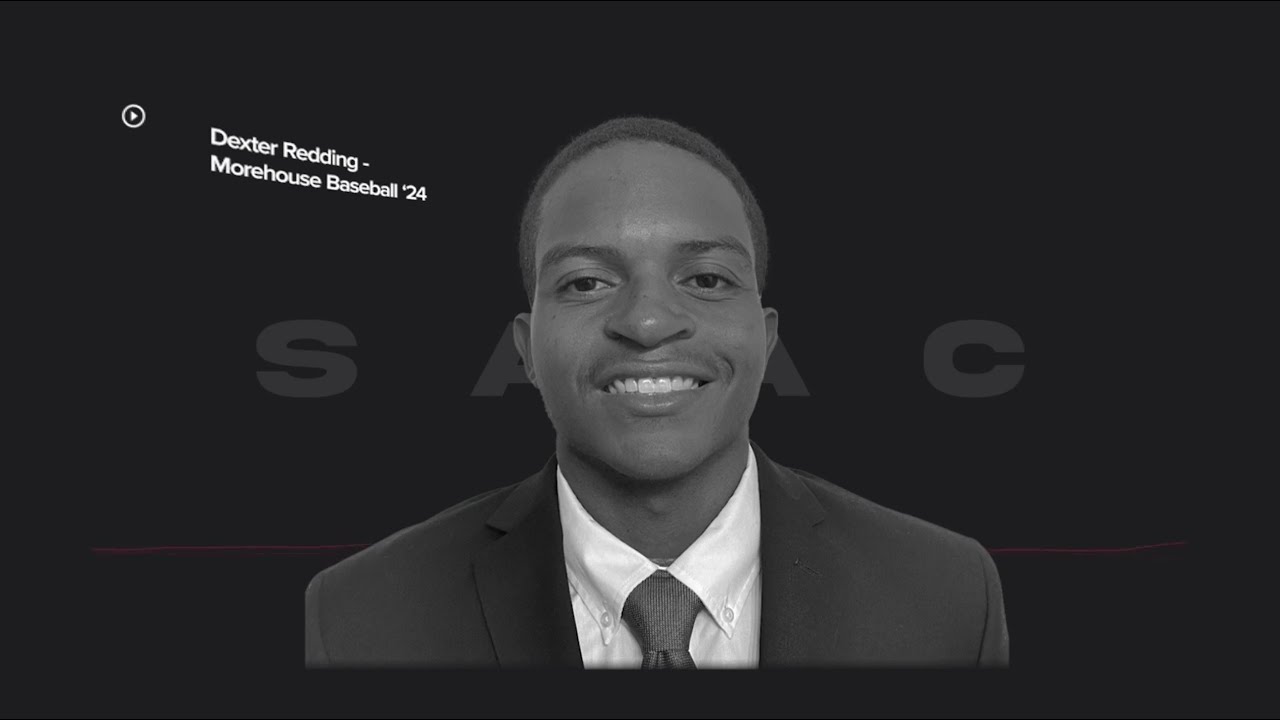The image features a professionally dressed man, Dexter Redding, who is the central focus, wearing a suit and tie, and smiling directly at the camera with a freshly groomed appearance. The backdrop is a plain grayish-black color with a watermark text overlay of "S A A C" partially visible behind his head. The top left corner displays text that reads "Dexter Redding, Morehouse Baseball 24," indicating his affiliation with the Morehouse College baseball team. There's also a small play button icon in the same corner. A thin red line runs horizontally behind Dexter's upper body, adding a subtle accent to the black and white photo. The image gives an impression of a formal headshot, likely for academic or athletic purposes, with a happy and enthusiastic expression from Dexter.